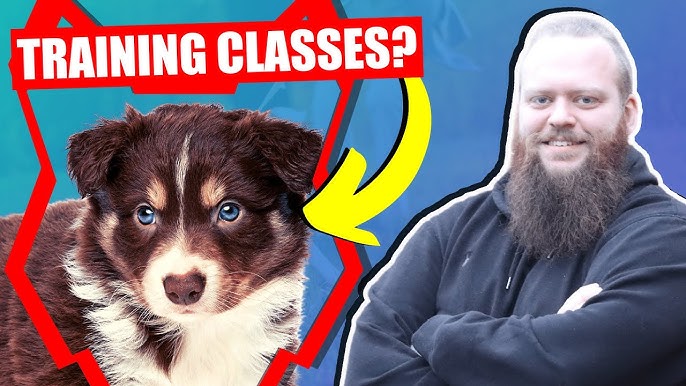The image, designed in a classic YouTube thumbnail style, features a smiling, heavier-set man with a big bushy beard and either short or no hair on his head, wearing a black sweatshirt, and standing on the right-hand side with his arms crossed. There is an aqua to dark blue gradient background. On the left-hand side, there is a small puppy with dark brown fur and white markings on its chest, between its eyes, around its little black nose, and under its fur, with striking blue eyes. The puppy is outlined by a red stylized dog shape, with a red rectangle at the top containing white text that reads "Training Classes?" A bright yellow arrow, outlined in black, points in an arc from the text towards the adorable dog's face. The overall design captures a vibrant and engaging contrast between the man and his small, expressive puppy, suggesting an inquiry about training classes.